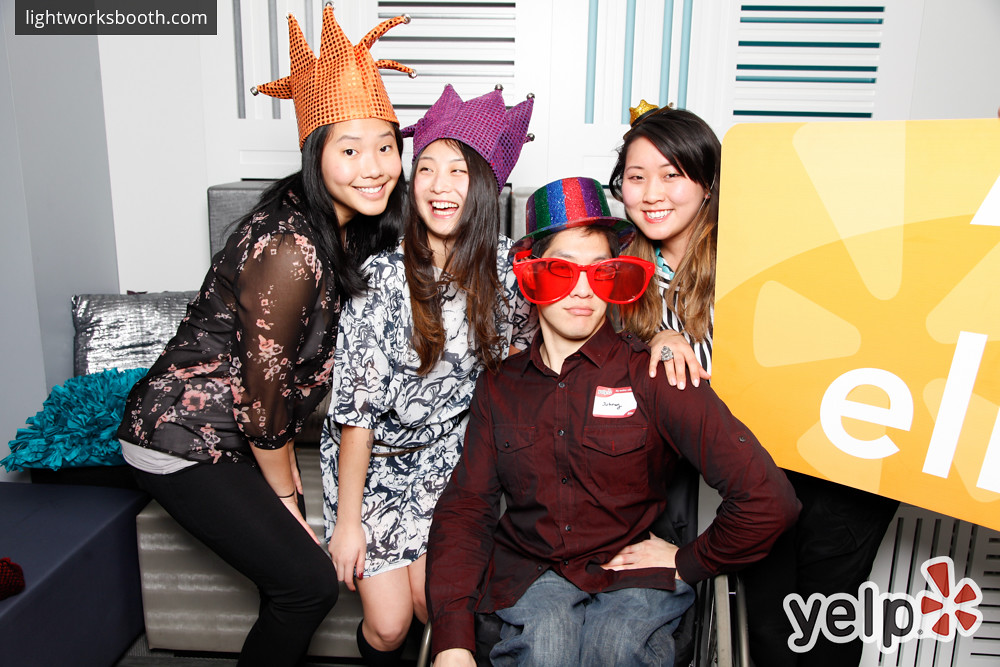This is an indoor, photographic image featuring four young Asian adults, professionally dressed for an event, highlighting the website lightworksbooth.com. In the foreground, a young man in a wheelchair dons a rainbow top hat, oversized red glasses, a purple collared shirt, and blue jeans. Next to him, on the left, is an Asian woman with shoulder-length black hair wearing a lacy black blouse with floral patterns, paired with black tight pants and an orange jester cap. Another woman, standing beside her, sports a purple jester cap, a black and white dress above her knees, and knee-high boots. Positioned to the far right is an Asian woman wearing a tiny, off-kilter top hat, a black and white striped shirt, and black pants. Her hand, adorned with a ring, rests on the man's shoulder. The backdrop features a mix of gray, black, white, and blue lines, suggesting a photo booth setting. Text on the upper left corner reads "lightworksbooth.com," and the bottom right corner displays a Yelp logo and partial letters "E-L-L" from a yellow and orange poster.